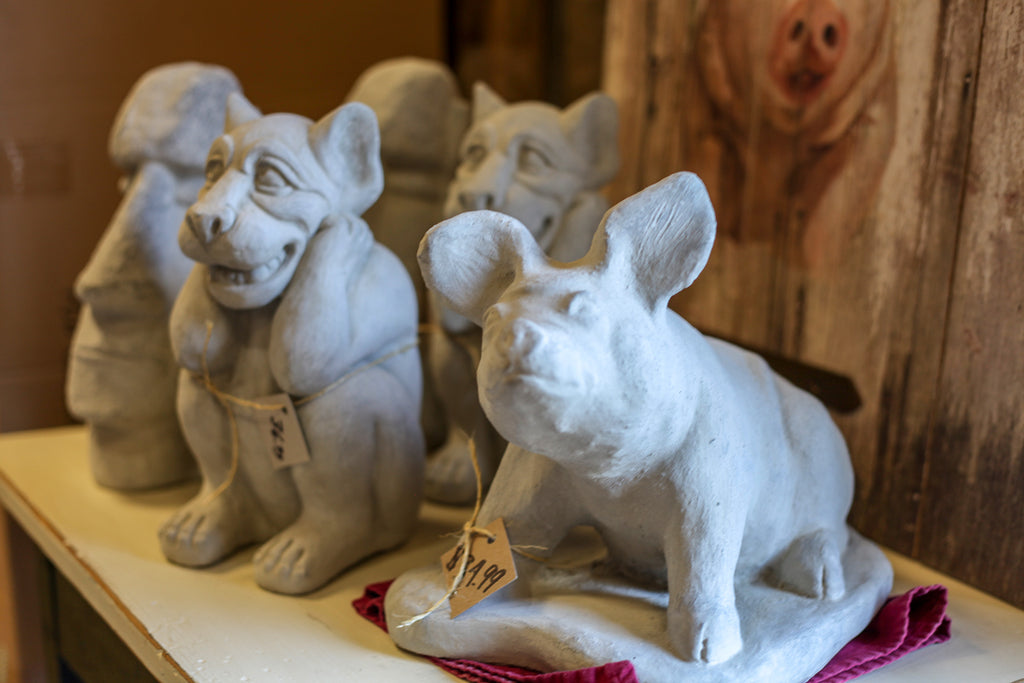This is a realistic and detailed photograph, horizontally oriented, showing five small sculptures arranged for sale on a white countertop in a store. The sculptures, unpainted and gray in color, appear to be made of materials like ceramic, concrete, or clay. In the foreground, there is a pig statue, approximately 12 inches tall and 12 inches wide, with a yellow price tag tied to its leg, marked $34.99 in black felt marker. This pig statue is positioned on a small red towel. Behind the pig are two gargoyle statues, each with distinct, ancient-looking features. Further back in the arrangement, two statues representing the iconic Easter Island heads stand impressively. The countertop is white, providing a clean backdrop for the sculptures, while a wooden wall forms the background. The image, albeit slightly zoomed in, makes the sculptures and their intricate details prominent, suggesting they are for sale in a store setting.